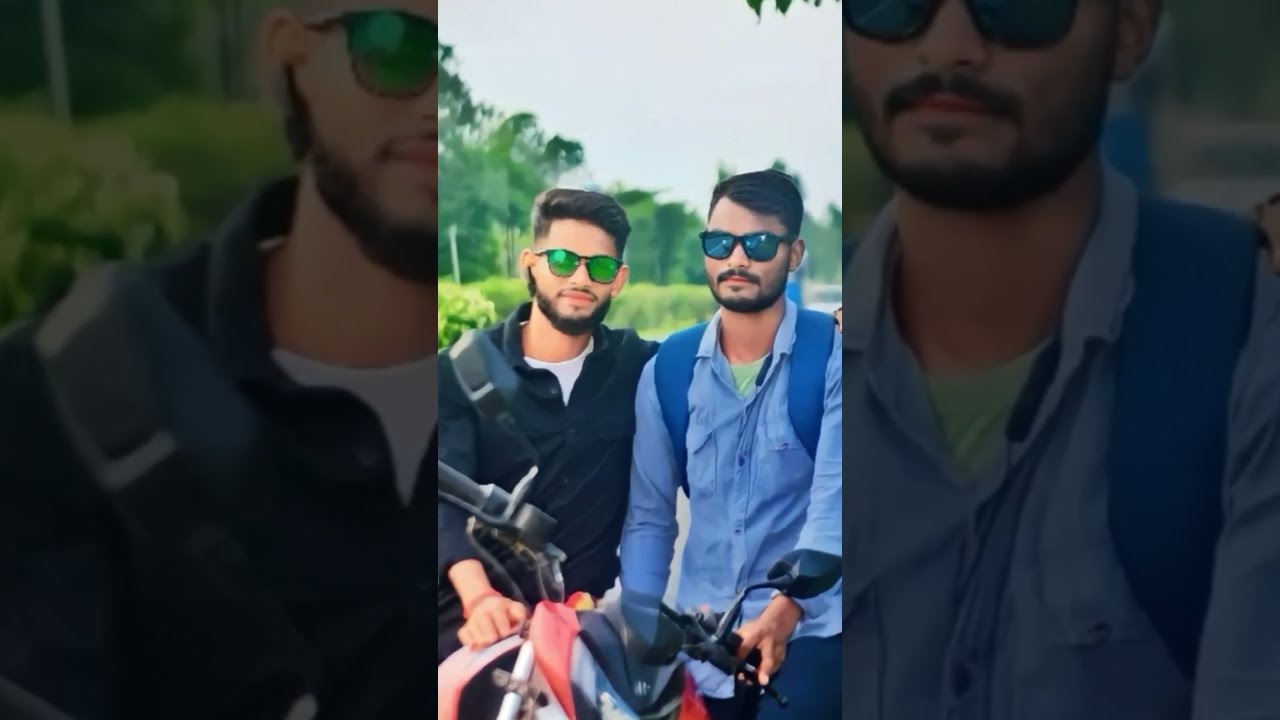In this detailed outdoor portrait photograph, we see two men in their mid-twenties centered in the image, posing side by side against a backdrop of green foliage and a gray-blue sky. Both men have neatly combed, short brown hair and wear sunglasses with colored lenses—one with blue lenses and the other with green. The man on the right sports a light blue button-up shirt over a green undershirt and a blue backpack. He has a thick dark brown beard and mustache and is holding the brakes or handlebars of a red motorcycle in front of him. The guy on the left, slightly behind the first, wears a dark blue button-up shirt over a white undershirt. His facial hair is medium-length and more concentrated around the jawline and neck. He also wears black sunglasses with green lenses and has his hand resting on the back of the motorcycle. The motorcycles, one red and the other black, are parked below them in the frame, complementing the overall color scheme of the image. The natural lighting captures the vibrant colors of their attire and the lush greenery behind them, adding to the portrait's vivid, outdoor setting.